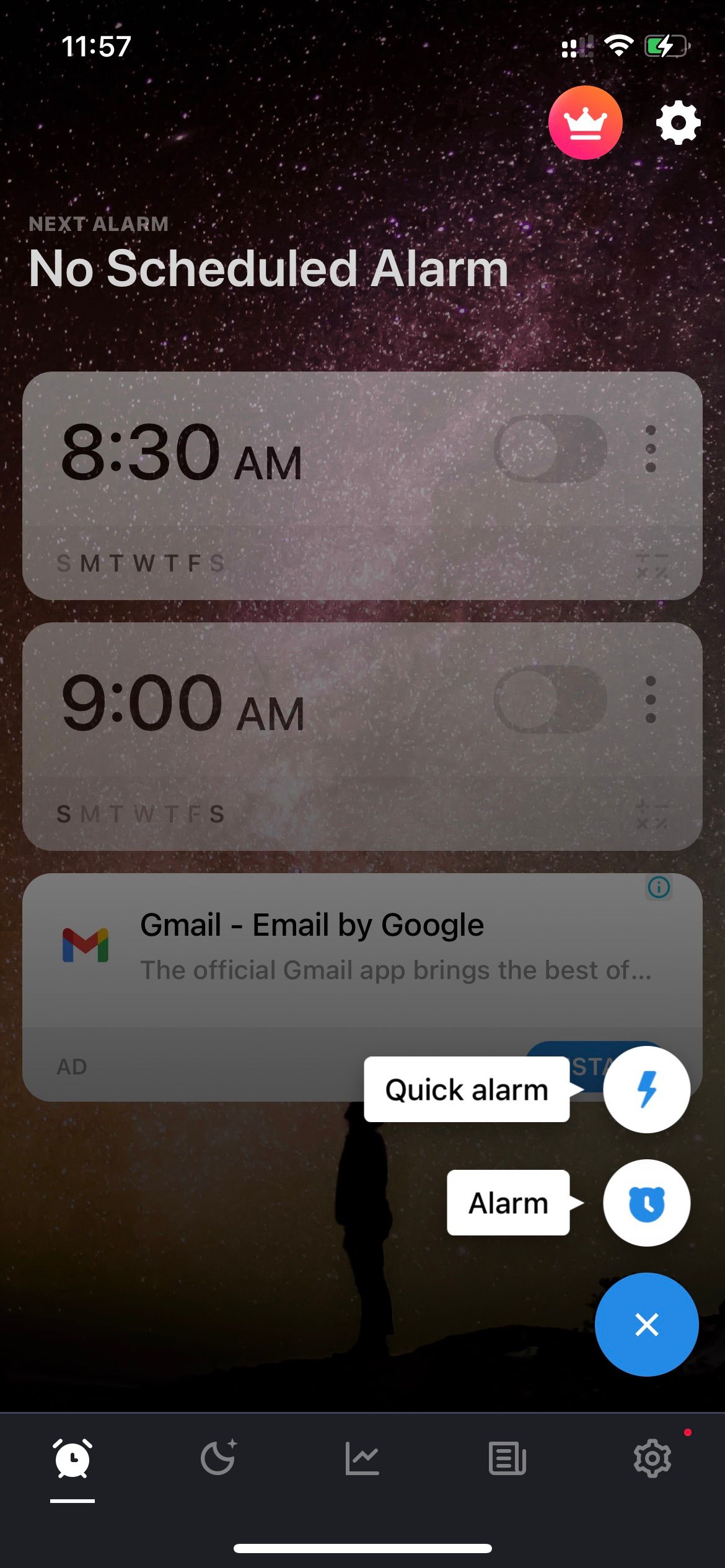Displayed on the screen of a smartphone is the time, prominently shown as "11:57" on the top-left corner, with indicators for cellular signal, Wi-Fi connectivity, and battery status on the top-right. The battery appears to be charging at around 50%. Just beneath these indicators, on the right, there's a circular icon in shades of orange and red, featuring a white crown within it, signifying an app or notification. Adjacent to this icon, there’s a settings gear icon.

Further down, the screen displays "Next Alarm" on the left in smaller white text, and below it, in a larger white font, it states "No scheduled alarm." Below this, there is a horizontally elongated rectangular box. Inside this box, it shows an alarm set for "8:30 a.m." followed by the days "Monday, Tuesday, Wednesday, Thursday, Friday, Saturday" indicated by their first letters in a row. To the right of this alarm, there is a gray toggle switch signifying it is off, and to the far right, three vertically aligned dots suggest more options.

Directly beneath this box, another white rectangle displays an alarm set for "9:00 a.m." with "Sunday and Saturday" noted. This second alarm is also toggled off, evidenced by the gray switch and the three vertically aligned dots for additional options on the right.

At the bottom portion of the screen, a message begins with "Gmail," followed by "Email by Google, the official Gmail app brings the best of..." and trails off with ellipses. In the lower-left corner, the word "Add" appears, presumably for adding more alarms or events.